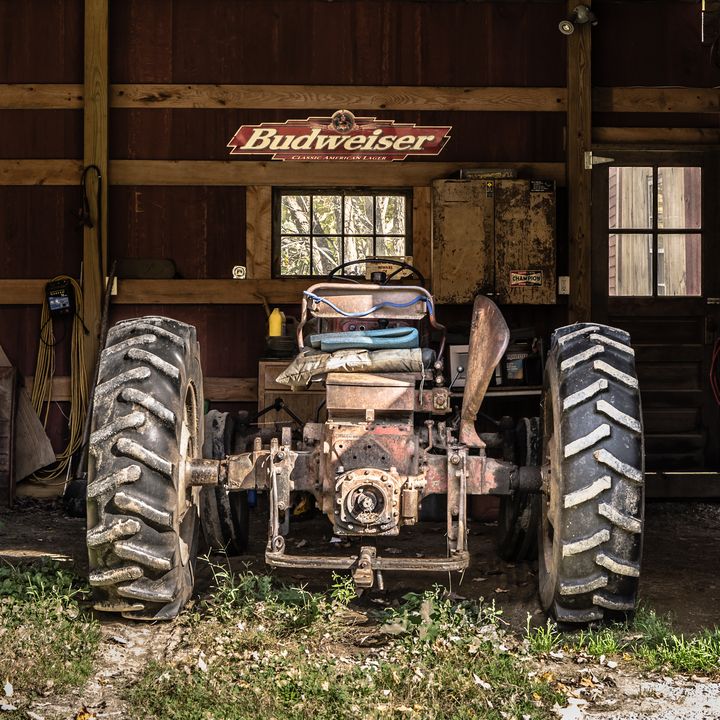The image depicts a close-up of an old, heavily worn-down tractor parked in front of a dilapidated wooden building, likely a barn. The rusted tractor, missing some metal parts, exposes its internal rivets and bolts, yet still has its black steering wheel intact. Its two large, very worn tires rest on a patch of grass and weeds with visible tire tracks. A cowboy boot is casually placed on the tractor, adding to the rustic scene. Behind the tractor, the weathered wooden wall of the building features a pale tan and brownish red Budweiser logo, and is adorned with various items including hoses or cords, a rusty metal toolbox, and a small light fixture in the right corner. Additional details such as a window, a door, a yellow bottle canister, and another indistinct sticker add to the sense of a space filled with heavily used, aged items.